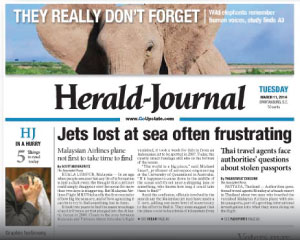In the image, we see the front page of a newspaper. Dominating the top left corner of the page are the words "They really don't forget" in white against a backdrop image of an elephant. The top half of the elephant is visible, facing directly towards the viewer, with light brownish-gray skin. The backdrop includes a blue sky and a green grass field.

Prominently centered in the newspaper, the text "To the right of that" is followed by the word "Tuesday" presented in blue. Beneath the newspaper's name "Herald Journal," we find additional text.

In the bottom left corner, a rectangular vertical image features a man in a black suit, with short black hair and a sad expression, rubbing his head. His skin is light-toned. Above this image, there is more text.

Lastly, to the right side of this image, an array of articles is present. One of the articles highlights a specific piece of information.